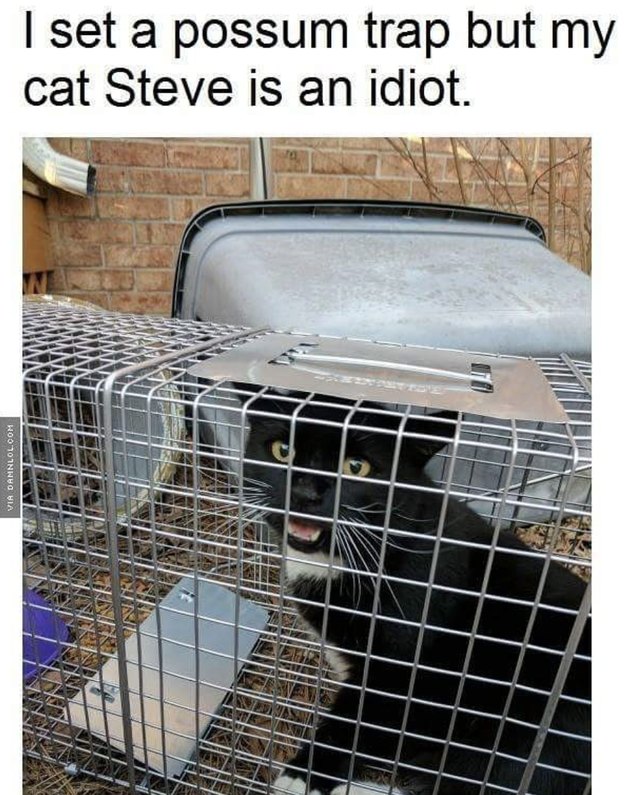The image displays a distressed black cat with some white fur on its chest and feet, trapped inside a silver possum trap. The trap is composed of thin bars and has a shiny silver plate on top. The cat is facing left with its yellow eyes wide open and mouth agape, revealing its pink tongue and white teeth. In the background, there is a tipped-over blue plastic container against a light red brick wall, held together with light gray mortar. To the left of the container is a spout. The scene is accompanied by black text at the top saying, “I set a possum trap but my cat Steve is an idiot."